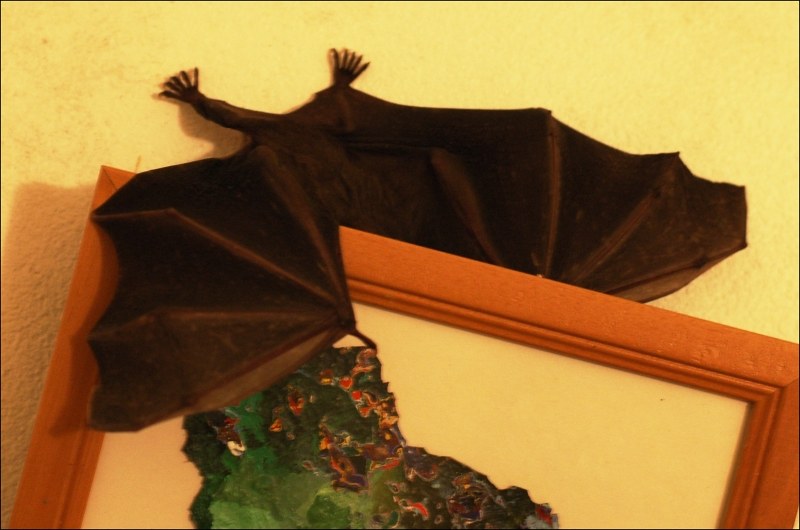In this image, a dark brown bat with its body and wings pressed flat against a pale yellow wall creates a stark contrast. Its two feet are prominently positioned up and to the left, appearing almost as if they are holding it in place. The bat itself covers a framed painting that features a vibrant green, red, and brown depiction, resembling an island or a dragon with an open mouth. The painting is housed in a decorative wooden frame with an orange or charred wood tone. The right wing of the bat overlaps the top of the picture frame, adding to the intriguing composition of the scene. The bat's head is obscured behind the frame, creating the illusion that it might be hiding or sneaking behind the artwork. Overall, the combination of the bat and the framed picture creates a fascinating and detailed visual story.